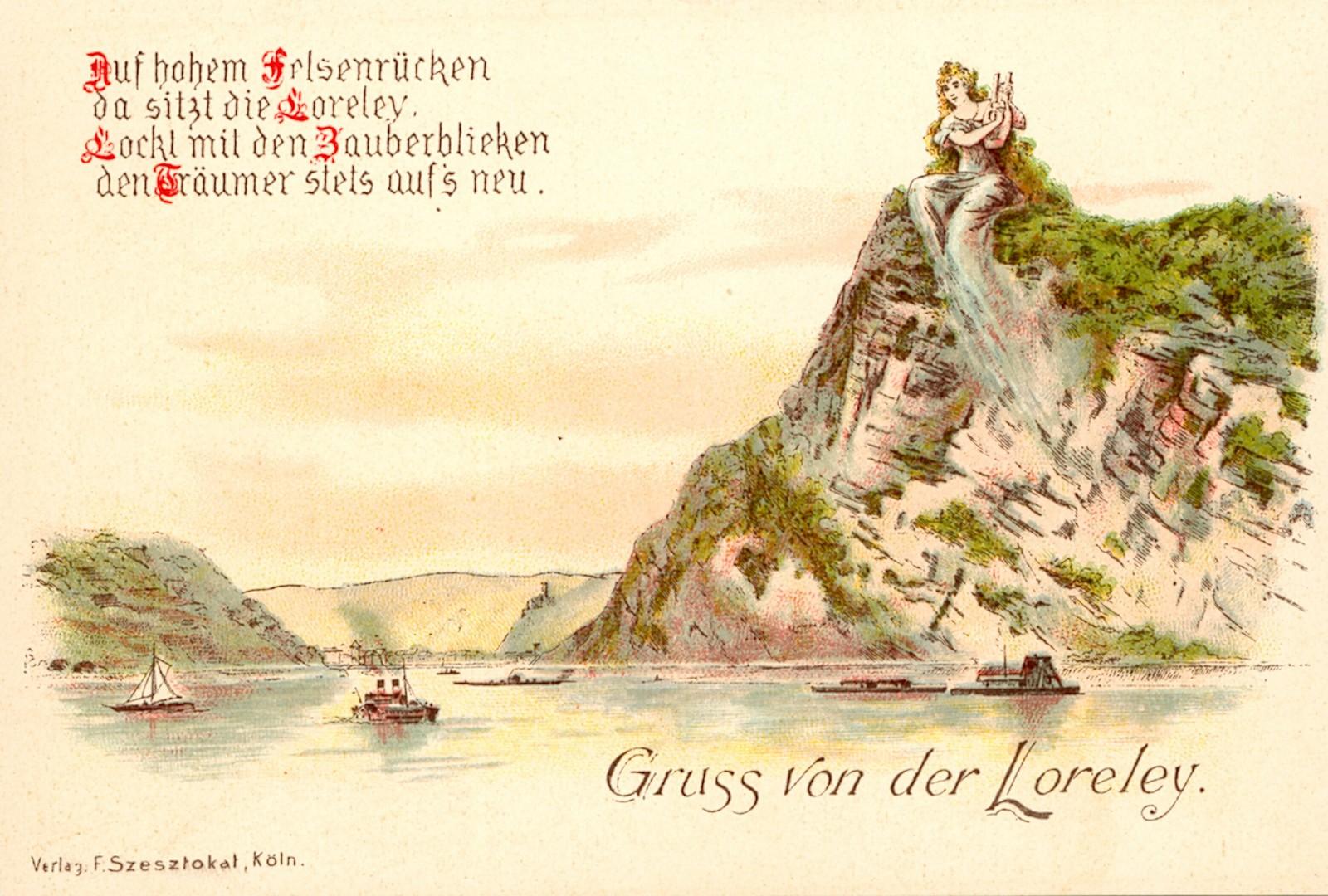The image is a detailed, hand-drawn scene likely intended as an advertisement or cover art, featuring a mythical or historical woman atop a large, mountainous cliff face. She is seated, wearing a greenish gown that seamlessly blends into the mountain itself, creating a natural, flowing effect. The woman, who appears to be white with blonde hair, is holding a harp or similar instrument. Below her, a serene seaside scene unfolds with several vessels navigating the water, including a steamship, a sailboat, and other boats. The mountain is depicted with abundant greenery, including shrubs and trees. The left side of the image features smaller hills, contributing to the overall natural landscape. The text, which is written in stylized German with capitalized red letters at the top left and black text at the bottom right, includes phrases difficult to fully decipher. Notably, the words "Gruss von der Loreley" are clearly visible, suggesting a greeting from Loreley, a legendary figure associated with the Rhine River in German folklore. The entire scene is bathed in a warm, possibly sunset glow, enhancing its mythical and inviting atmosphere.